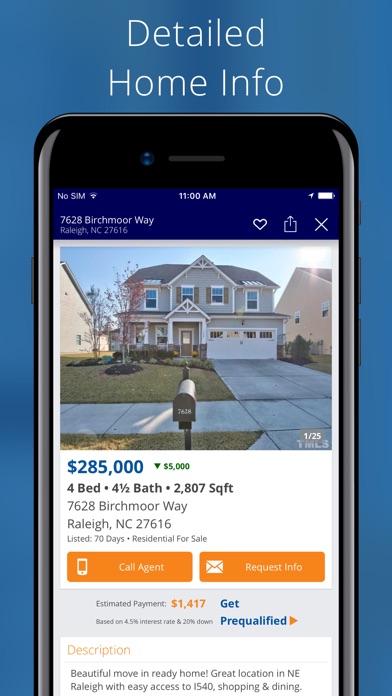The image features a blue background with the centered white text "Detailed Home Info" in a thin-lined sans-serif font. A partial image of a smartphone is visible in the frame, displaying the top section of the phone screen. The screen shows a dark navy banner with "No SIM" in the upper left corner, an icon of a dot with a line over it, the time "11:00 AM," a send icon, and a battery icon. Below the banner, the address "728 Birchmore Way, Raleigh, North Carolina 27616" is prominently displayed.

In the lower part of the screen, there are icons for a heart, a share/send function (depicted with a square and an arrow above it), and a close button (an X). The smartphone screen shows an image of a house taken on a sunny day, with the sun visible in the right-hand corner. The house has a white exterior with darker tan trim and overall appears gray. It is a two-story structure with a single front door. The center of the image highlights the mailbox.

At the bottom right corner of the smartphone screen, text indicates "1 of 25 images," suggesting a gallery of photos. The house is listed for $285,000, showing a recent price drop of $5,000. Additional details include "4 bedrooms," "4.5 baths," and "2,807 square feet," each marked with a bullet point.